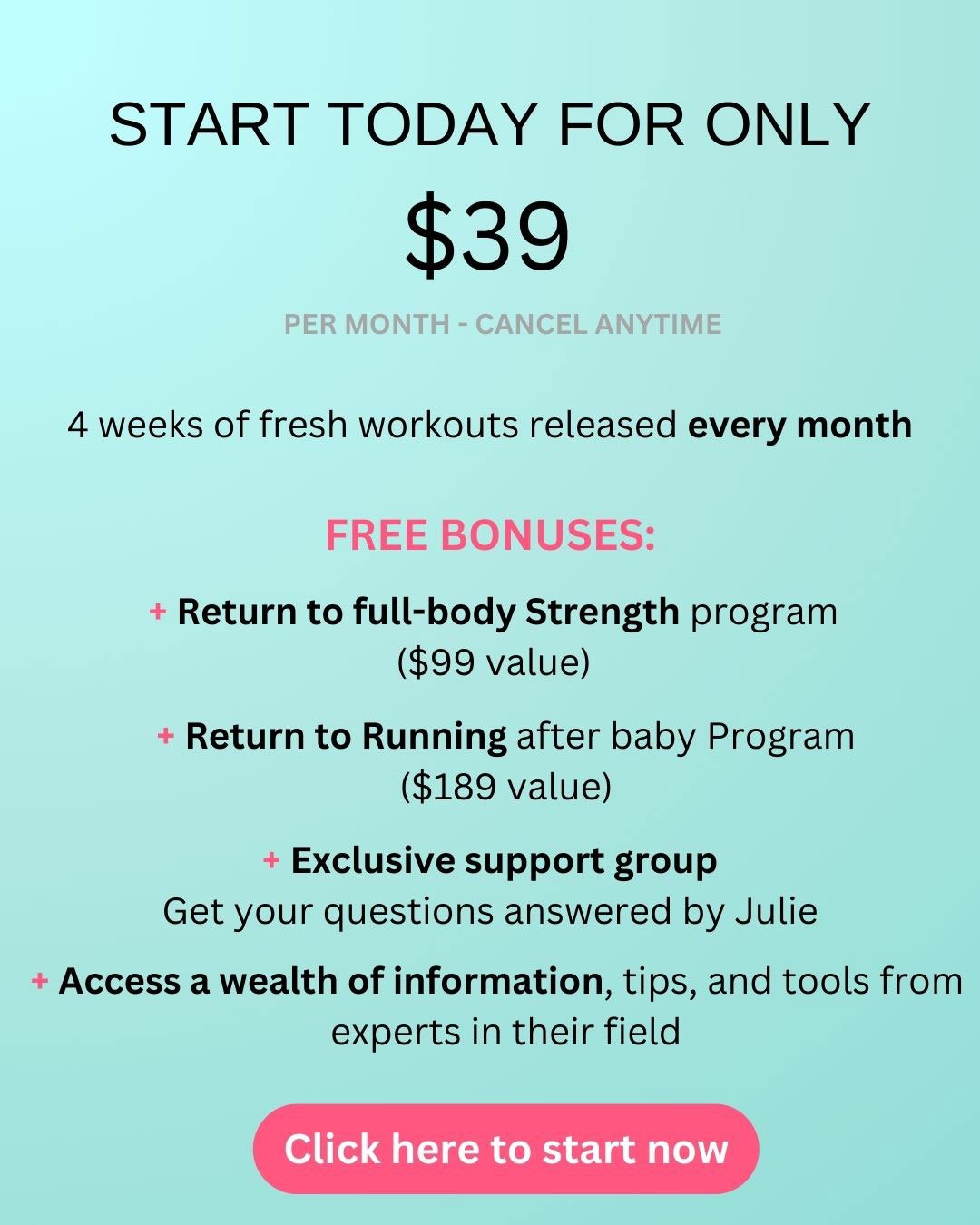The image features a digital banner with an aquamarine background and various pieces of text in different colors and sizes. The banner's headline reads "Start Today for Only $39" in bold, black letters. Below this, in smaller grey text, it states, "per month, cancel anytime."

A "Free Bonuses" section is prominently displayed with the heading in vibrant pink. This section lists four points, each marked with a pink cross or plus sign instead of traditional bullet points. The points are:

1. "Return to Full Body Strength Program" - a $99 value
2. "Return to Running After Baby Program" - a $189 value
3. "Exclusive Support Group: Get your questions answered by Julie"
4. "Access a wealth of information, tips, and tools from experts in their field"

At the very bottom of the banner is a prominent "Click Here to Start Now" button in hot pink, with the text in white.